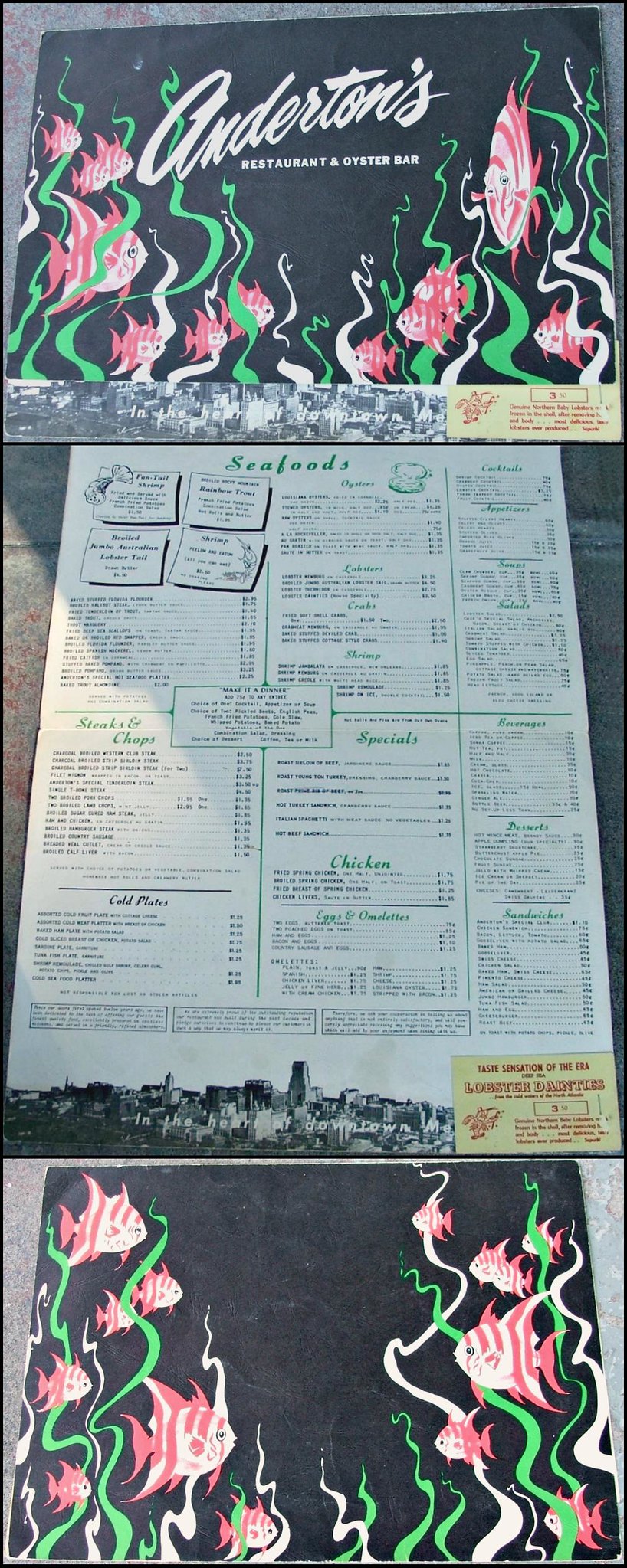The image is a vertical collage composed of three distinct photographs. The top section showcases a restaurant sign adorned with a fancy, cursive font stating "Anderton's." Below the main text, the subtext reads "Restaurant and Oyster Bar." The sign features artistic illustrations of fish, enhancing its nautical theme.

The middle section of the collage displays a close-up of the restaurant's menu. It appears to be a single-page menu titled "Seafoods," fitting for an oyster bar. The menu includes an array of options such as chicken dishes, daily specials, cocktails, and cold plates.

The bottom section presents what looks like a chalkboard menu, likely positioned outside the restaurant to attract patrons. The chalkboard retains the whimsical fish illustrations seen on the primary sign but omits the "Anderton's" branding and subtext. The background is predominantly black, typical of a chalkboard used for daily specials or announcements.